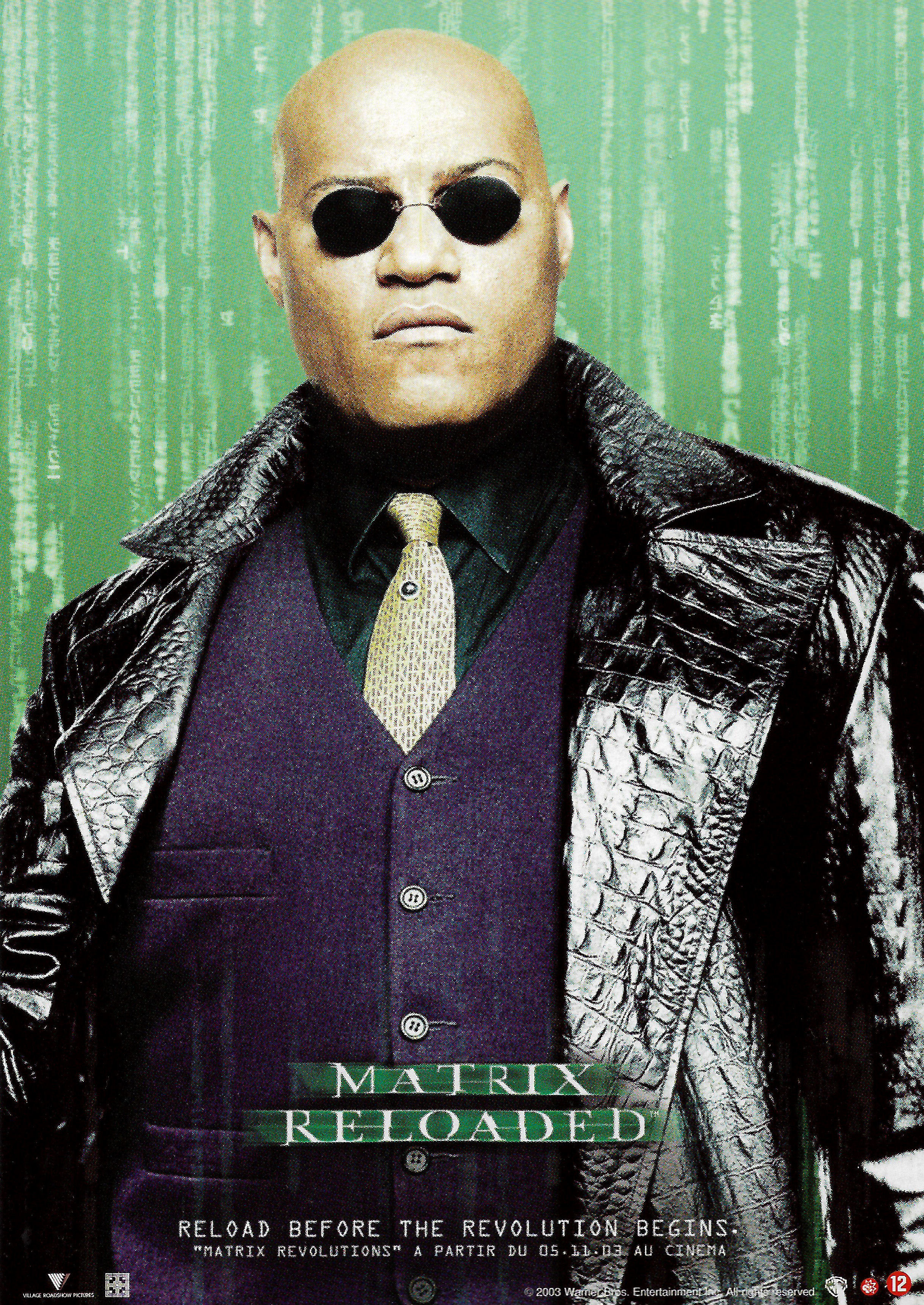The image is a detailed movie poster for "Matrix Reloaded" featuring the upper body of a stern-looking African-American man with a shaved head, wearing dark, oval sunglasses. He is dressed in layered attire, which includes a black button-down shirt complemented by a gold tie, underneath a fully-buttoned purple vest with plastic purple buttons. Over this, he sports a distinctive black leather jacket that has a textured, reptilian-like finish. The backdrop is a greenish hue adorned with vertical white streaks, giving the impression of raindrop-like stripes. At the midsection of the poster, the title "Matrix Reloaded" is prominently displayed in white letters with a green shade. Beneath this, the text reads, "Reload Before the Revolution Begins. Matrix Revolutions. Apartheid Due 05-11-03 AU Cinema." At the bottom, it includes the small print, "2003, Warner Brothers Entertainment, All Rights Reserved," along with a tiny WB logo.